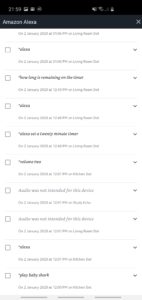This image is a blurred screenshot from a smartphone, featuring a predominantly white background with a black top border. Despite the poor quality and lack of focus, certain elements are discernible. In the upper left-hand corner, against the nearly black background of the top border, there appears to be "Amazon Alexa" written in a grayish-white font. Above this text, small icons indicating battery status and wireless connection strength are visible. Below this section, the main screen displays a lengthy list of items, each written in a gray font. To the left of each item, there is a gray box, which might suggest an option for selecting or checking off the item. On the right side of each item, there is an inverted triangle icon, hinting at the presence of a drop-down menu for additional options or settings.